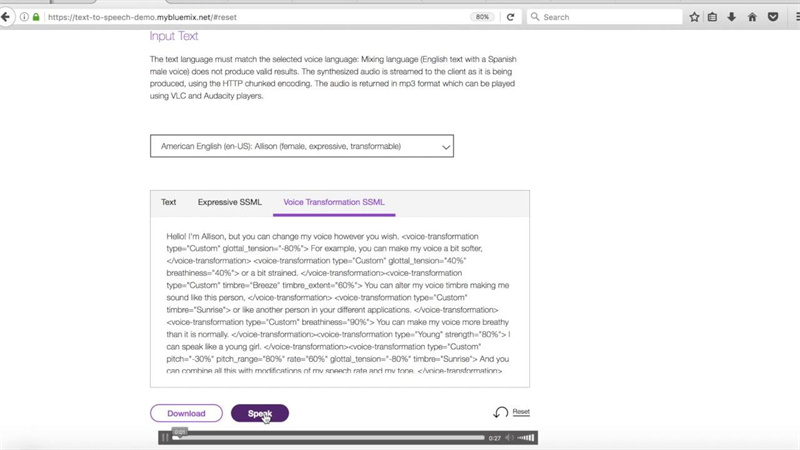This screenshot captures a web page hosted at the URL `text-to-speech-demo.mybluemix.net/#/reset`, visible within a browser window with a silver-gray background. The web page itself features a white background. At the very top of the page, in gray font, the text says: "Input text. The text language must match the selected voice language. Mixing languages (e.g., English text with a Spanish male voice) does not produce valid results. The synthesized audio is streamed to the client as it is being produced using the HTTP chunked encoding. The audio is returned in MP3 format, which can be played using VLC and Audacity players."

Below this explanatory text, there is a drop-down menu set on a white background, displaying options for selecting the language and voice. Currently, it shows "American English (US) - Allison (Female, Expressive, Transformable)". Further down, there is a section dedicated to inputting text, featuring a rectangular text box. The section header is displayed against a light gray background and reads "Text (Expressive SSML: Input Text)", with a sub-section header highlighted in purple, "Voice Transformation (SSML: Transformation)".

Beneath the text box, two buttons are visible: on the left, a white button labeled "Download" and on the right, a purple button with white font labeled "Speak". At the very bottom of the page, there's a small audio player interface, offering the option to play the synthesized audio sample directly.